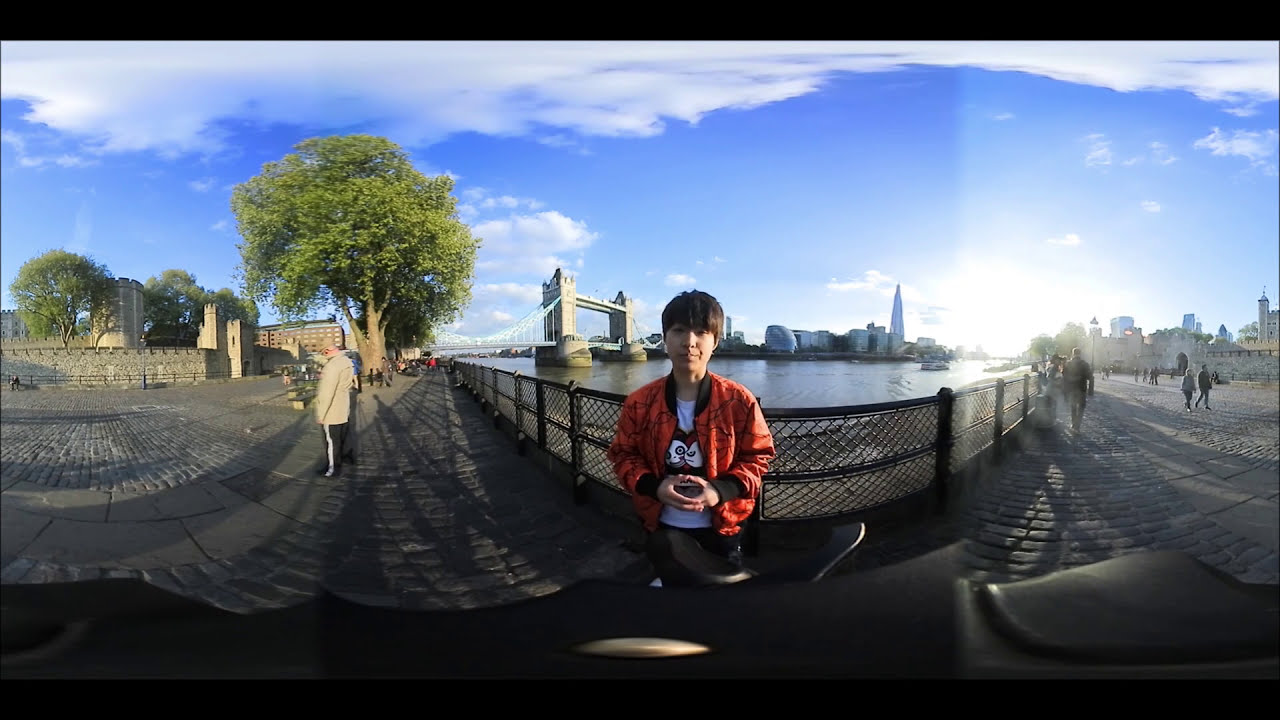A panoramic photograph shows a young Asian man, possibly in high school or college, standing on a stone or cobblestone boardwalk next to a large river. The path beneath him is composed of a stone or brick surface. He is visible from the waist up and is wearing black pants and a white graphic t-shirt depicting two cartoon characters looking at each other. Over the t-shirt, he sports an orange-red jacket with a black collar and black wrist cuffs, which is unzipped. His hands are in front of him, playing with his fingers.  

In the background, to the left of his head, is a large suspension bridge while a city skyline is visible to the right. Behind him is a black metal railing with a chain-link fence, separating pedestrians from the river. The sky is a bright blue, spotted with a few white clouds, and trees with vibrant green leaves are to the left of the photograph. There are also indications of a few boats on the water. The scene appears to capture a historic, well-maintained, and architecturally interesting area, likely a tourist spot.